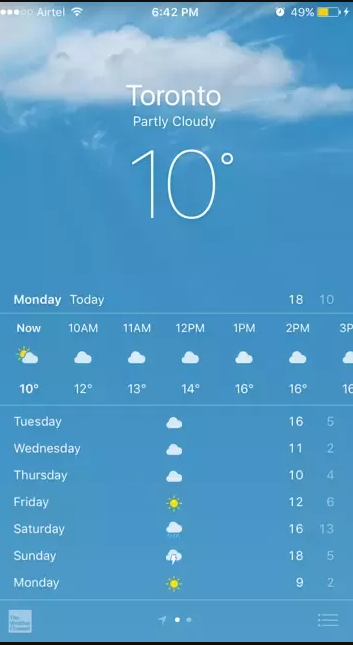The image depicts a weather forecast interface for Toronto, presented in a highly organized and detailed manner. At the top, the interface displays various phone status indicators: signal strength on the left, the current time (6:42) in the middle, an alarm icon, and a 29% battery life indicator. 

Prominently featured in the upper-middle section is the weather forecast for Toronto, highlighted in bold. The condition is noted as "partly cloudy" with a significant temperature display of "10°C" in a notably large font size. Adjacent is an illustration of a few puffy clouds against a blue sky, representing the current partly cloudy weather.

Directly beneath this, the word "Monday" is bolded, indicating the day of the forecast. Under the "Monday" label, it reiterates "10°C" with a partly sunny icon and details of weather conditions from 10 AM through 3 PM. These hourly updates show corresponding temperatures and an icon depicting partly sunny to cloudy conditions.

To the right of "Monday," the word "Today" is displayed, signifying the day's forecast. Below this section, there are columns providing a week-long outlook. These columns include the days of the week, weather conditions (sunny or cloudy), high temperatures, and low temperatures.

At the bottom of the screen, a small thumbnail indicates that the weather information is provided by The Weather Channel. Additionally, a pagination indicator shows three dots, with the second dot highlighted, indicating the user is on the second page of the forecast. In the bottom right corner, three horizontal lines suggest a menu option where users can add or delete cities for weather updates.